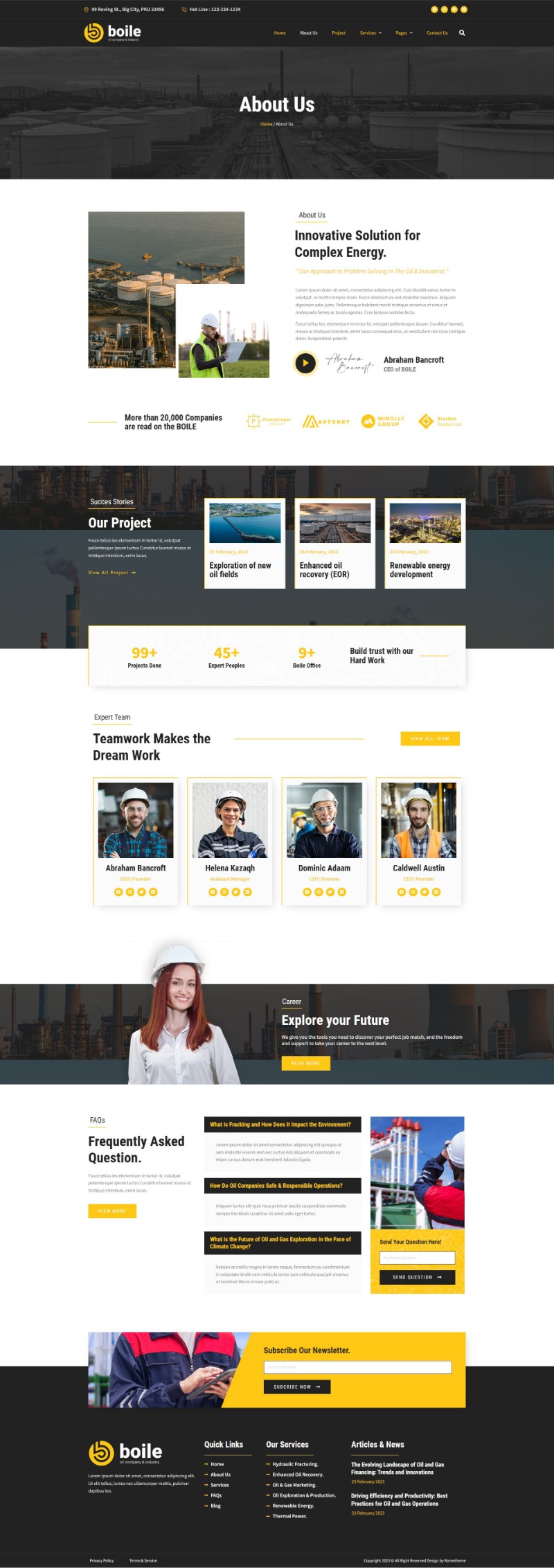This image is a detailed screenshot of a webpage titled "About Us" for Boyle, a company operating in the energy and oil industry. The header section includes a top bar at the very top, providing the company's address, "99 Roving Street, Big City, PKU 23456," on the left side, and a hotline number, "123-234-1234," on the right, labeled as "Hotline" with a phone icon. Below this, the navigation bar features the company logo, "Boyle," along with the tagline, "Energy and Industry," prominently displayed on the left. The navigation links are listed as Home, About Us, Projects, Services, Pages, and Contact Us, with a search icon located at the far right of the navigation bar.

The main content of the page highlights a hero section, which includes a large banner with a background image depicting an industrial site. Centrally placed in the banner is the title "About Us" in large white text. Below the title, breadcrumb navigation is shown, indicating the path as Home > About Us.